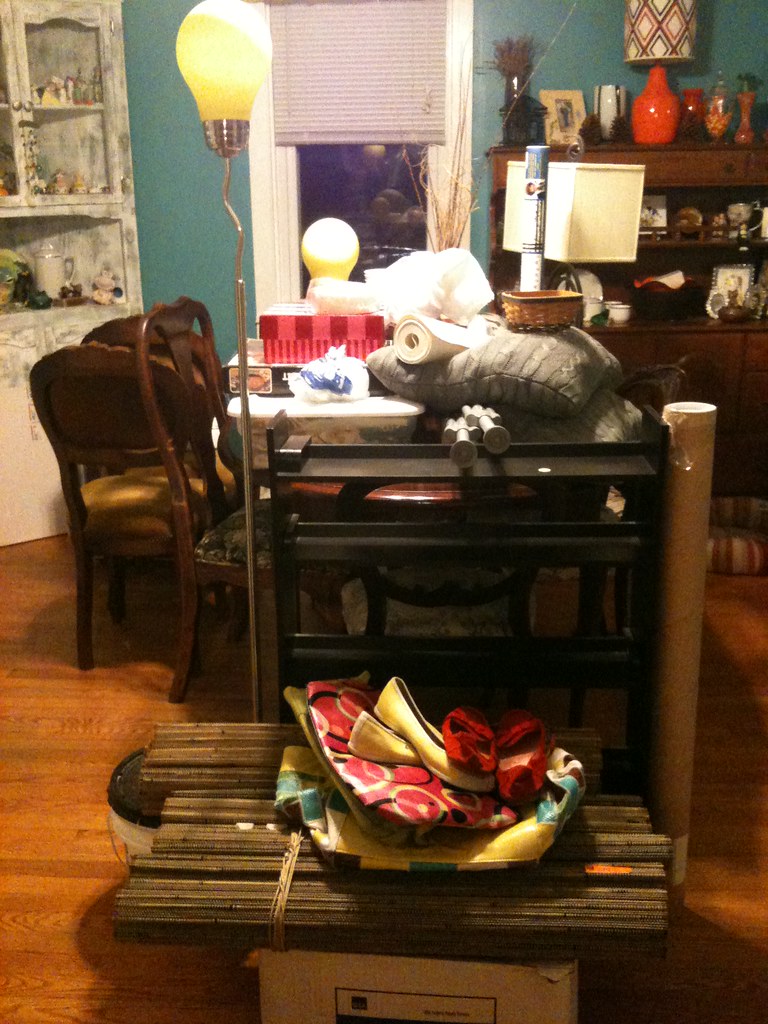The image depicts a dining room with a richly detailed interior. On the left-hand side, there is a marble-finished white cabinet, likely used for storing dishes. It is adorned with a white pot and several smaller decorative items. The backdrop of the room features green, black, brown, and yellow cabinets, complementing a bluish-green wall. A window with horizontal plastic shutters is visible, which are raised about halfway up.

Central to the scene is a table cluttered with various items. Behind this table, a yellow and white spherical light fixture hangs, partially obscured. On the table, a red and pink box sits atop another box, which features an image on it, accompanied by a white and blue plastic bag in the foreground. Cushions are stacked with a small basket placed on them. 

The room contains wooden chairs and a pair of yellow and white light bulbs on a gold stand. Several lamps are visible in the background, including one with a square, cream-colored shade and another with a round, red and black patterned shade with a matching red base. These lamps rest on another wooden cabinet that holds more items, such as a jar of dried plants and a framed photograph.

In the foreground, another cabinet is seen with a gray object on it, positioned in front of the table. On top of a cardboard box nearby, there are bits of wood, colorful bags in shades of green, yellow, red, and black, as well as pairs of yellow and red shoes. The overall scene suggests a lively, well-used space filled with a mix of functional and decorative elements.